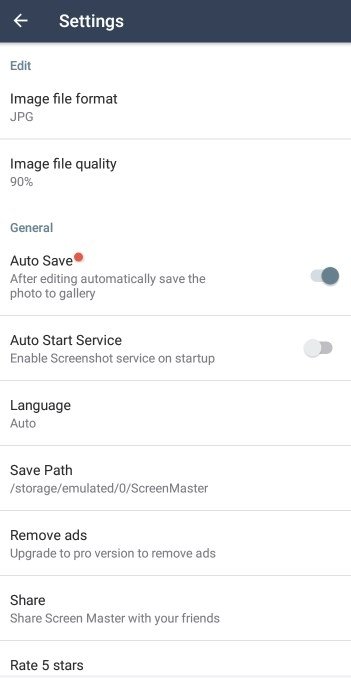The image showcases the settings screen of the "Screen Master" app, presumably designed for capturing and sharing screenshots. The interface is predominately white with black text. At the top, there is a navigation bar with a "Back" button that allows users to return to the previous page.

Several settings are detailed on this screen. First, the image file format is set to JPEG, with the file quality adjusted to 90%. There is an 'Auto Save' toggle, which is turned on, indicated by a red dot next to it—possibly an edit to guide users. The 'Auto Start Service' is off. The language setting is set to 'Auto detect.' The save path is specified as "storage/emulated/0/Screen Master," suggesting where the screenshots are stored.

Below these options, there is a button to remove ads by upgrading to the pro version. Users are also encouraged to share the app with friends and rate it five stars.